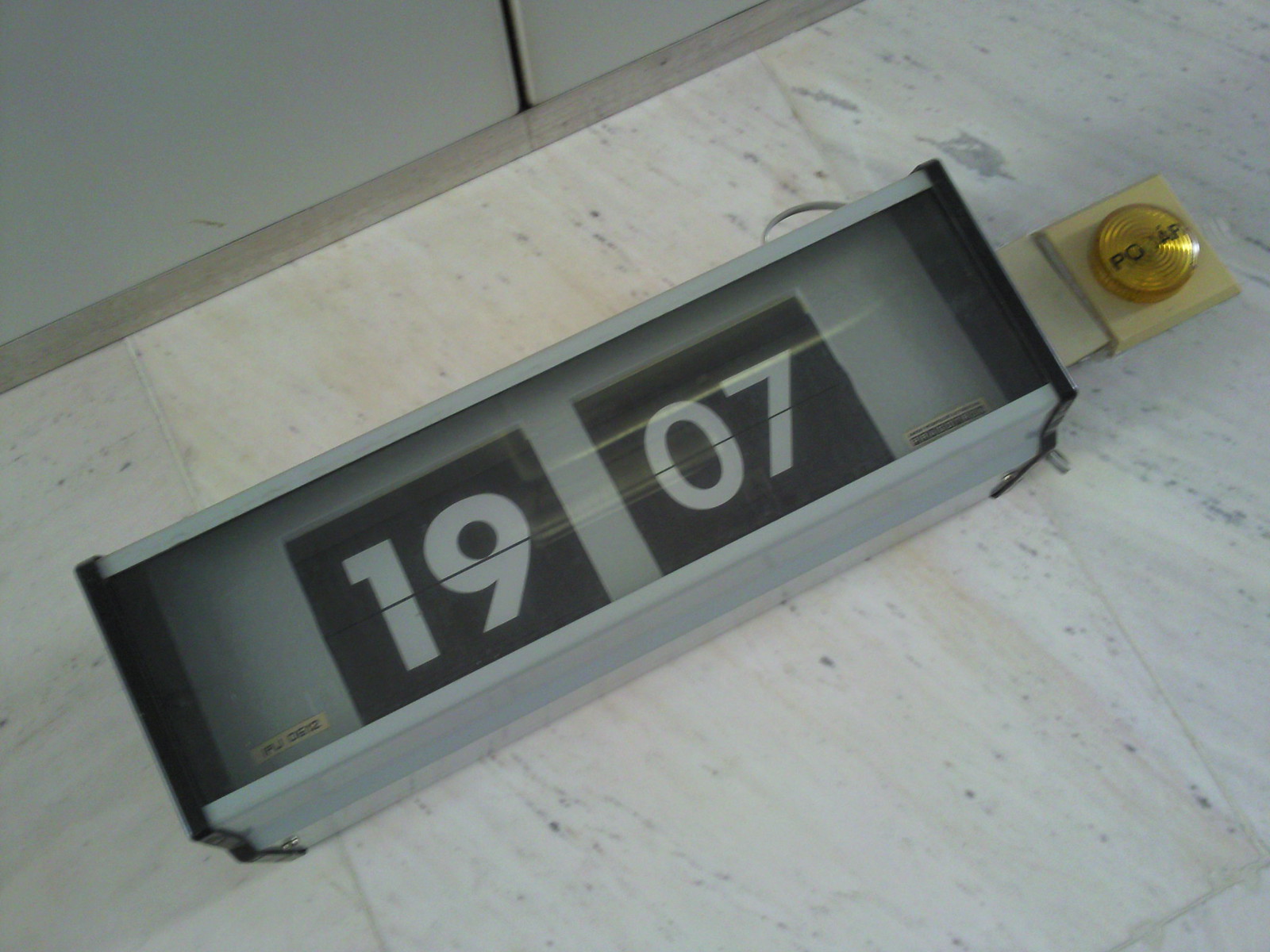This photograph features an analog flip clock resting on a tiled floor. The clock is housed in a sleek, metal gray rectangular casing, and its display currently reads "19:07." Instead of a digital display, this clock uses rotating cylinders to show the time. A thin line runs through the center of the time display, indicating where the numbers should align. Next to the clock, there is a button labeled "P-O." The overall setting seems to be well-lit, highlighting the modern yet retro design of the clock against the clean, tiled backdrop.